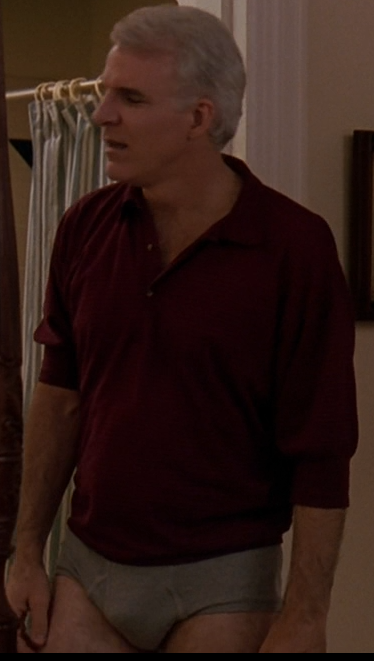This is a detailed photograph of the actor Steve Martin, likely captured from a scene in a movie. Steve Martin, an older white male with prominently gray hair, is seen standing upright and looking to the left. He is dressed in a dark reddish, unbuttoned long-sleeve shirt, exposing part of his chest. He sports classic gray tighty-whitey underwear, a comedic wardrobe choice frequently seen in films. Behind him is a partially opened shower curtain, indicating that the setting is a bathroom. The background also features a yellow and white painted wall, along with a framed item—possibly a photo or painting—hinting at a domestic environment. Steve Martin’s mouth is open as if he’s mid-sentence, suggesting he is engaged in conversation.